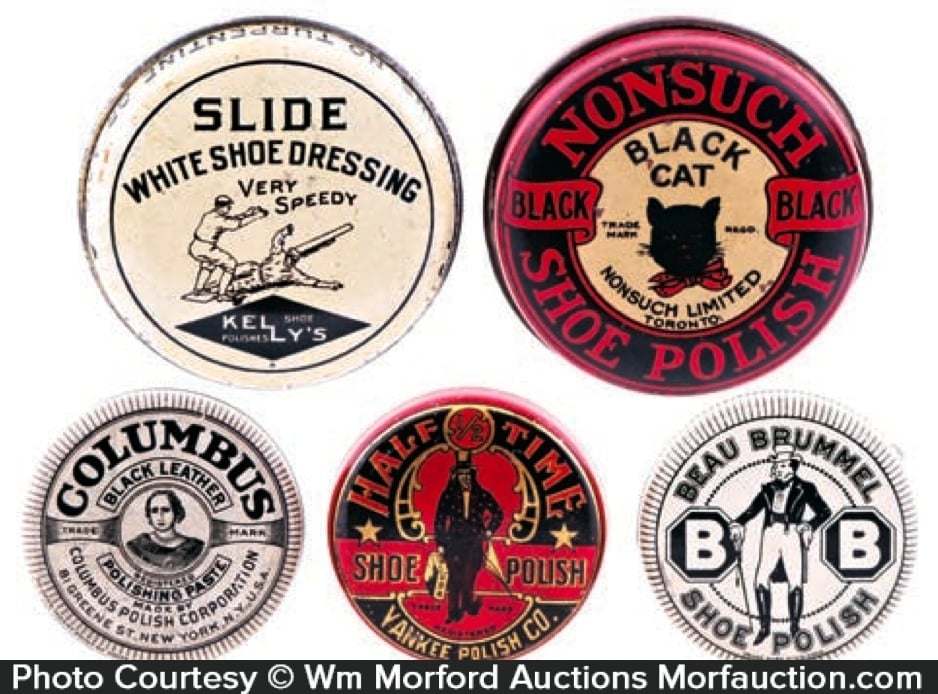This image showcases a collection of five vintage shoe polish tins against a white background. At the bottom of the image, a black text bar features the white font, "Photo Courtesy W. M. Morford Auctions, MorphAuction.com." The tins are arranged with two larger ones at the top and three smaller ones along the bottom. The top left tin is white with black lettering and depicts two baseball players, labeled "Slide White Shoe Dressing, Very Speedy." The top right tin is primarily red and black, featuring an illustration of a black cat and the words "Non-Such Black, Black Shoe Polish." 

On the bottom row, the leftmost tin is black with red lettering, stating "Half Time Shoe Polish by Yankee Polish Company," and displays an image of a man. The middle tin is white with black lettering, portraying a portrait and labeled "Columbus Black Leather Polishing Paste." The rightmost tin is also white and features the text "Beau Brummel Shoe Polish" along with an illustration of a well-dressed gentleman from the 1800s holding a cane. Each tin varies in color and design but collectively reflects the branding and artistry typical of historical shoe polish products.